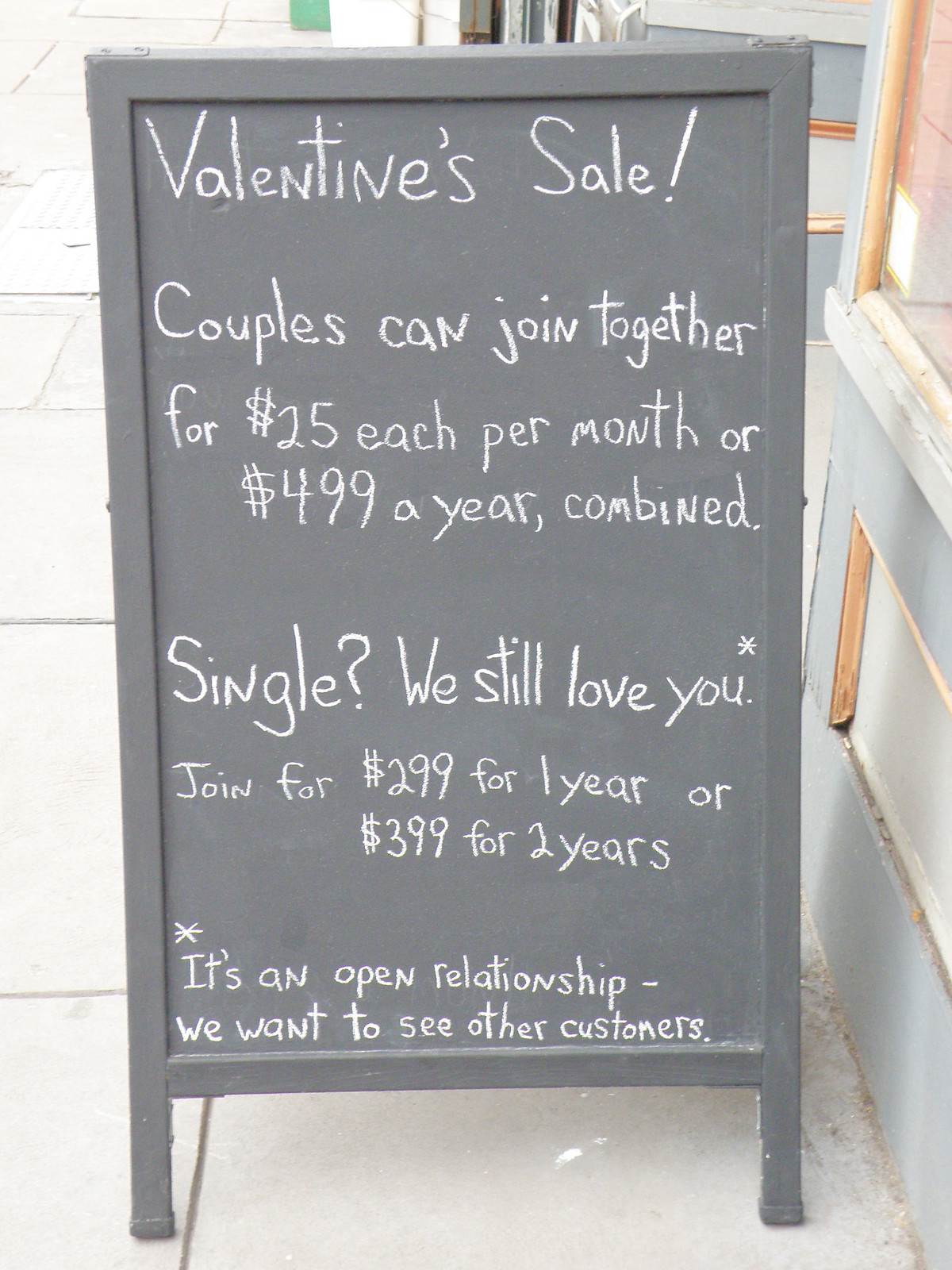The image depicts a black, fold-out chalkboard stand placed on the sidewalk outside a shop, promoting a Valentine's Day sale. The sign, written in white chalk, offers a romantic-themed promotion with details for both couples and singles. It reads: "Valentine's Sale! Couples can join together for $25 each per month or $499 per year combined. Single? We still love you! Join for $2.99 for one year or $3.99 for two years.*" An asterisk at the bottom playfully remarks, "It's an open relationship. We want to see all the customers." The shop, located to the right, features a gray and gold facade with a window frame at the top right. The image is taken during the daytime, with the sidewalk visible on the left and bottom sides.